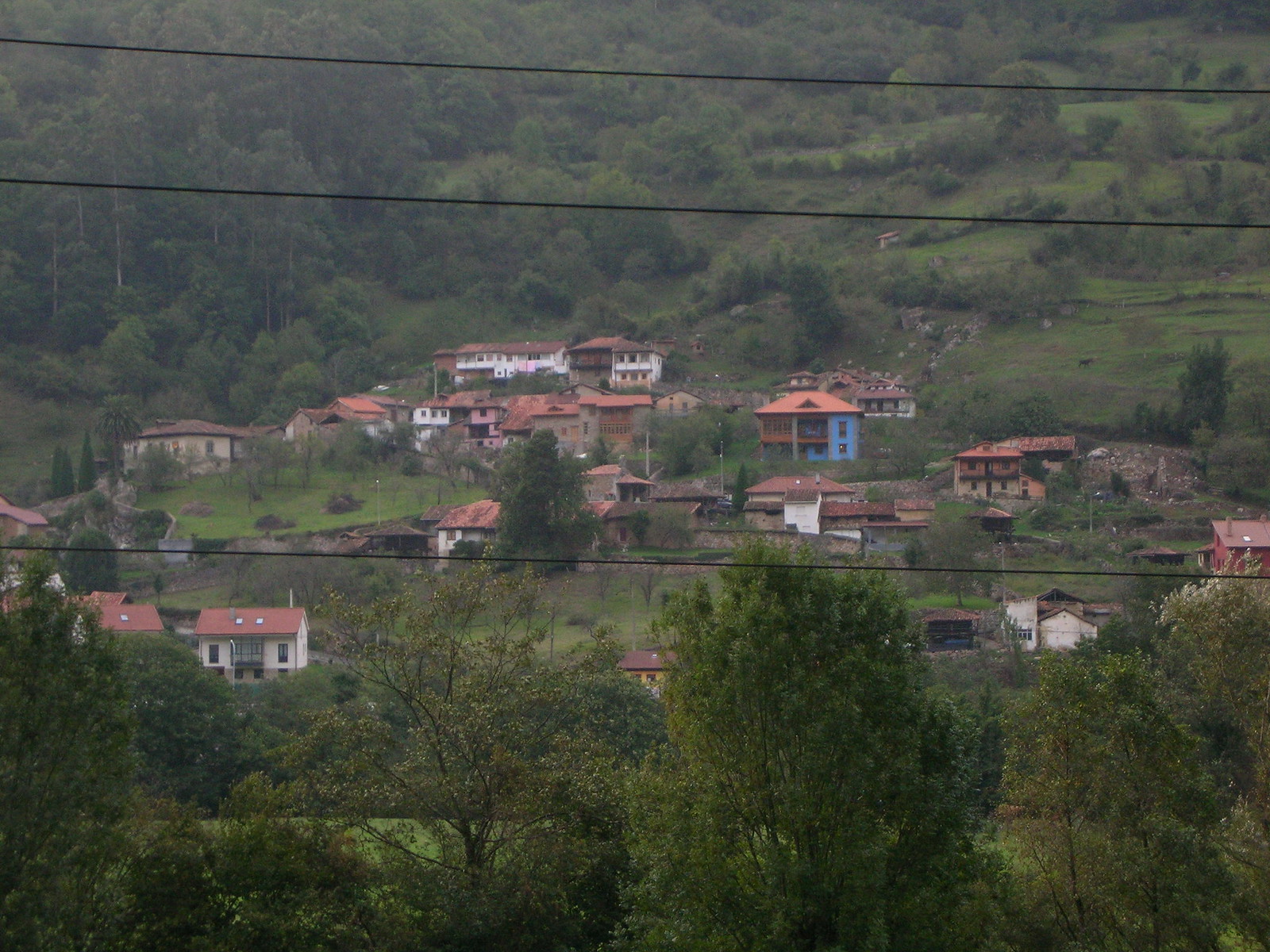The photograph captures a distant town perched on a sloping hillside, which descends from the top of the image towards the bottom. The hill is adorned with numerous species of trees, all lush and green, giving the impression of a dense yet open forest surrounding the town. The town itself is comprised of multiple multi-storied buildings, predominantly featuring white exteriors with red roofs. One central building stands out with its unique half-brown, half-blue facade. Although the buildings appear somewhat worn, they add character to the scenic landscape. Visible in the foreground are three black power lines running horizontally from left to right. The overall scene is bathed in daylight, enhancing the vibrant greenery and the quaint charm of the hillside town.